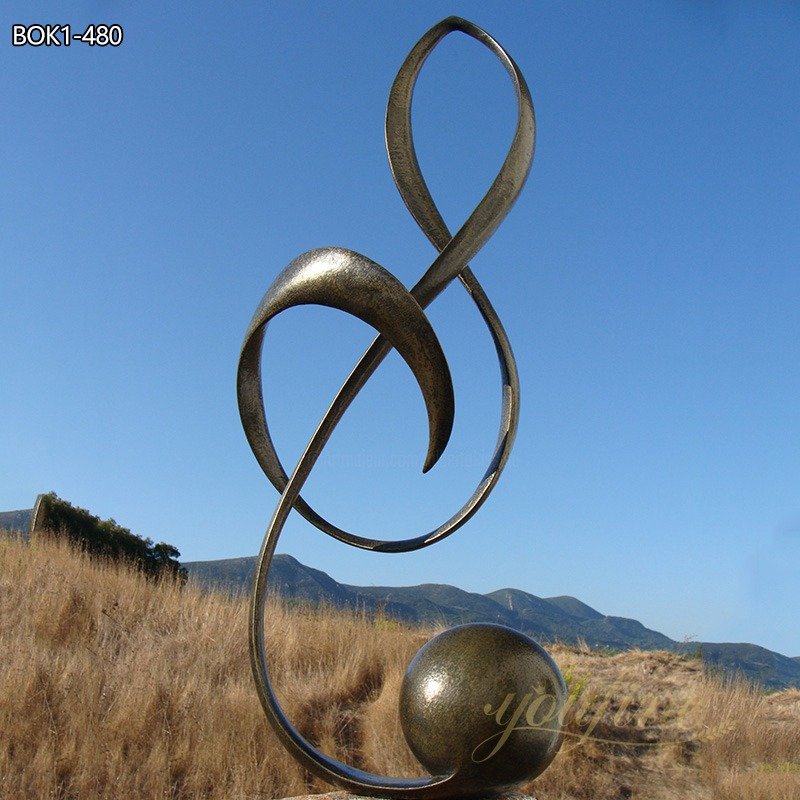This square photograph captures a modern metal sculpture set against a vast, outdoor prairie landscape, with dry grass stretching across the terrain and distant mountaintops visible under the expansive blue, cloudless sky. The artwork, constructed possibly from bronze or steel, features a large, heavy metal ball at its base. From this, a sinuous, curving line ascends gracefully, forming what resembles a G clef—an iconic musical notation symbol. The artist's name, "YOUJINE," is inscribed in gold lettering in the lower right corner, indicating the creator of this striking, contemporary piece.